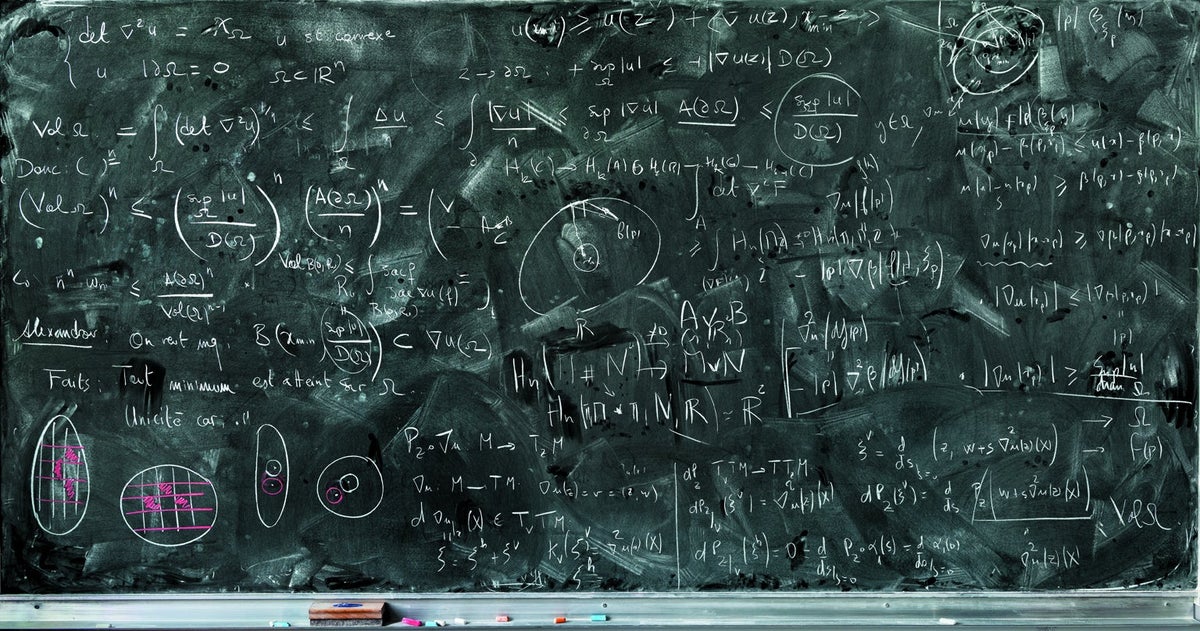This image captures a heavily used, dark green chalkboard entirely covered with dense algebraic and scientific notations, extending from one side to the other without any empty space. Along the bottom edge, the metallic chalk tray holds an eraser and multiple small pieces of chalk in various colors, including pink, blue, orange, and white. In the lower left corner of the chalkboard, some colorful chalk drawings add a splash of pink, with shapes resembling circles and ovals, one featuring a grid-like pattern. The overall texture of the board reveals a history of numerous writings and erasures, evidenced by its smudged and dirty appearance, blending green and white hues in a chaotic manner that would be intelligible only to those well-versed in mathematics or science.